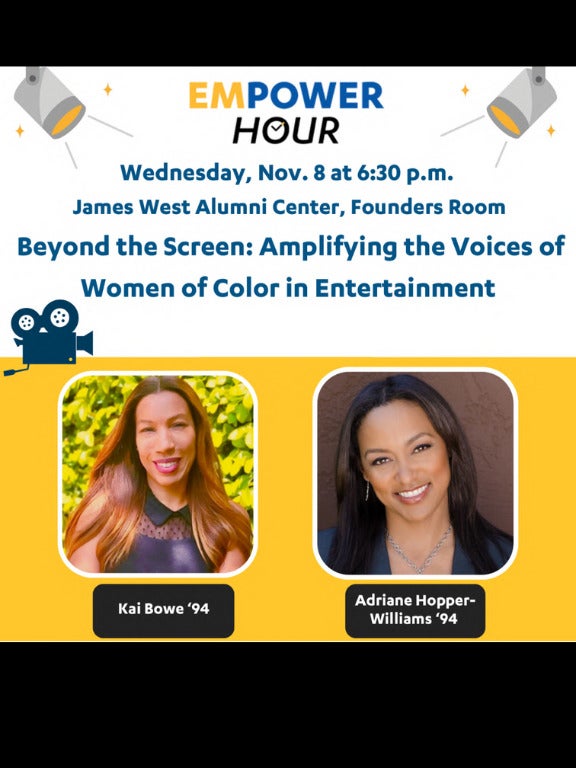This is an advertisement flyer for an event called Empower Hour. The top of the image features two flat vector stage spotlights shining down on text that reads "EM" in gold letters, "Power" in dark blue, and "Hour" in black, with the "O" designed like a clock with two hands. Below this, additional text in blue states the event details: "Wednesday, November 8th at 6:30 PM, James West Alumni Center, Founders Room. Beyond the Screen: Amplifying the Voices of Women of Color in Entertainment." A small black TV camera icon is positioned to the left of the text.

The bottom of the image has a gold background featuring real photographs of two women in square frames. On the left is Kai Bow, class of '94, smiling in a sleeveless black shirt with a green bush or plant background and light brown hair. On the right is Adrienne Hopper Williams, class of '94, also smiling, with long dark brown hair, a black top, a silver necklace, and drop earrings, set against a dark brown background. This section is framed by a black bar at the bottom of the flyer.